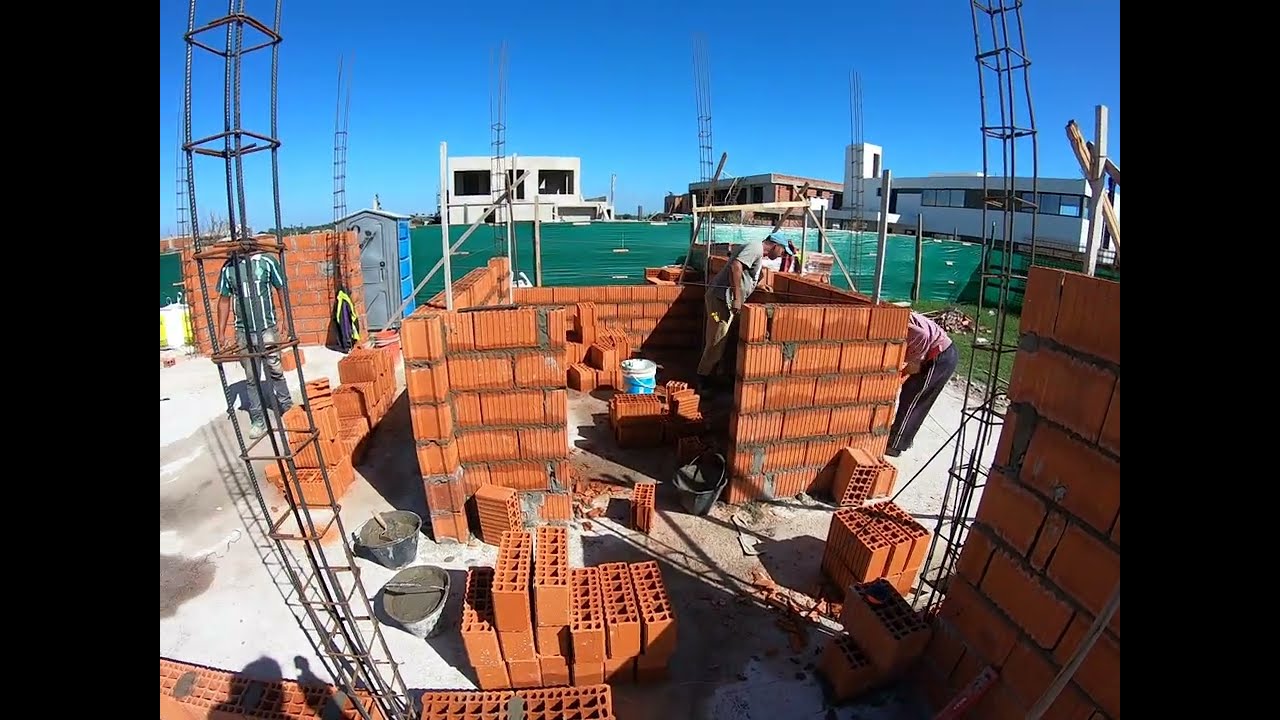The image depicts a bustling construction site where a group of men, likely masons, are diligently constructing a small, semi-square building out of reddish-orange clay bricks. These bricks resemble cinder blocks in shape but have a distinct red hue. The structure currently stands about four feet high, with the workers carefully stacking the bricks and applying mortar to secure them. Some rebar columns are visible on the left and right sides, providing additional reinforcement. In the foreground, there are stacks of unused bricks ready to be incorporated into the evolving structure. Surrounding the construction area is a green plasticky fencing, signaling that this zone is designated for construction activities. Beyond this fencing, several buildings are visible; some of them are covered in stucco cement and glass, mirroring the style of the new structure. One white building with windows, appearing complete, can be seen to the right. The overall scene captures the collaborative effort and meticulous process involved in building the small brick edifice, set against the backdrop of an active construction environment.